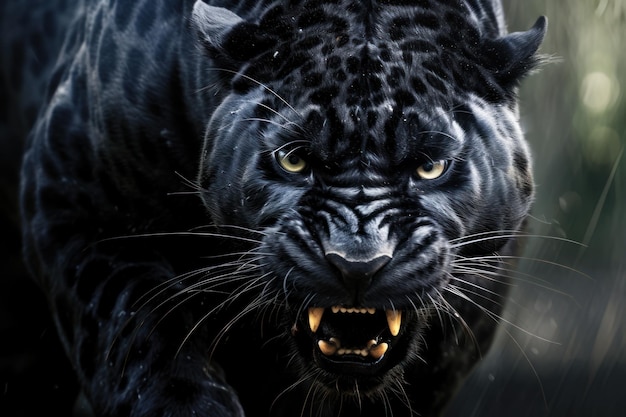This is a detailed digital close-up photograph of a large, menacing black panther or possibly a jaguar, seemingly in the midst of an attack. The panther's jaws are wide open, showcasing its sharp, yellow teeth with black tips at the ends. The menacing expression is heightened by its greenish-gold eyes and numerous prominent white whiskers. The panther is primarily black, with hints of gray and subtle black spots visible on its back, legs, and head. The background is predominantly black and blurry, with a little white ball of light, adding an eerie contrast to the scene. The overall composition focuses intensely on the panther, which is depicted with a snarling, aggressive stance, making the image appear charged with imminent danger.